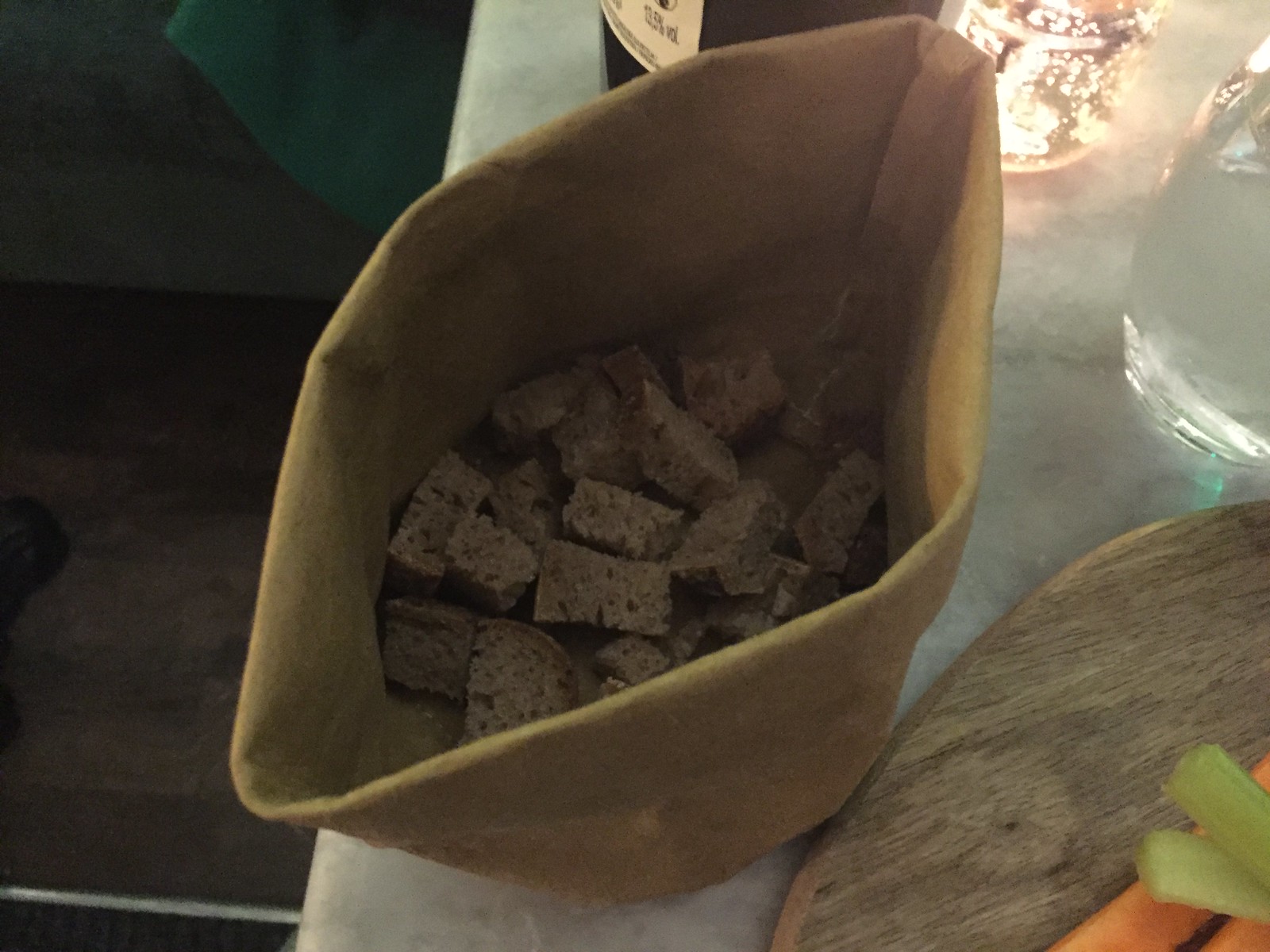The image is a color photo with a gentle, filtered light, presenting a table setting from a top-down perspective. Central to the composition is a deep, light brown cloth-lined basket filled with small, cubed pieces of brown bread, devoid of crusts and without any perforations, suggesting a dense, rustic wheat or rye texture. Adjacent to the basket on the bottom right is a brown, wood-grained serving board, meticulously arranged with two celery sticks and two carrot sticks set perpendicularly to each other.

In the upper right quadrant of the photo, a glass pitcher of water, beaded with condensation, stands tall next to a clear glass filled with sparkling liquid. To the left of the glass, partially visible, is a dark bottle with a label, hinting at champagne or mineral water. Also in the upper right corner, there's a candle in an open holder, casting a soft, ambient light over the scene. The items rest on a light-colored surface, possibly a stone table, and the left side of the image features a darker, indistinct background. A glimpse of what appears to be the tip of a toed sock suggests a human presence near the scene.